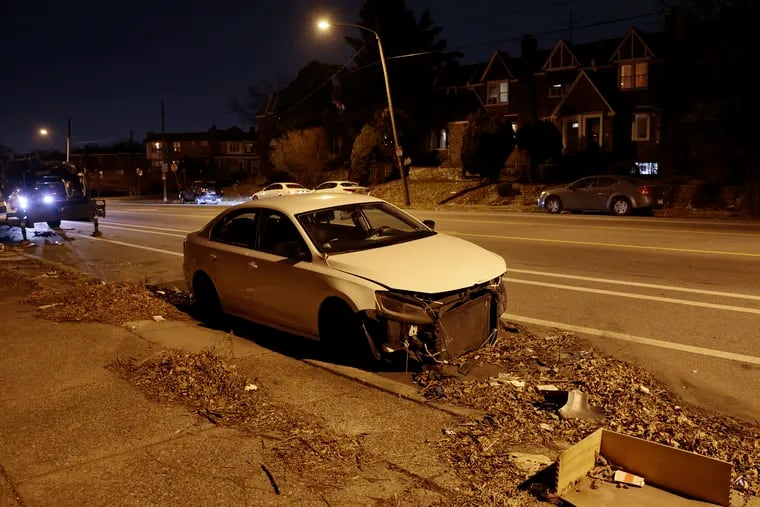A nighttime street scene featuring a white, four-door sedan parked along the street. In front of the car, the pavement is strewn with dirt, leaves, and assorted garbage. On the sidewalk adjacent to the car, there is half of a cardboard box containing various items. Scattered pieces of debris, possibly remnants from an accident involving the car, are evident on the ground. The image is somewhat blurry toward the front, adding to the chaos and mystery of the scene. The street itself appears to be multi-laned, with another car in the background displaying its headlights. Several other vehicles are parked across the street, and one of them also has its headlights on. Across from the cars, residential houses line the street, mostly dark with only a few showing lights from within, emphasizing the late hour.